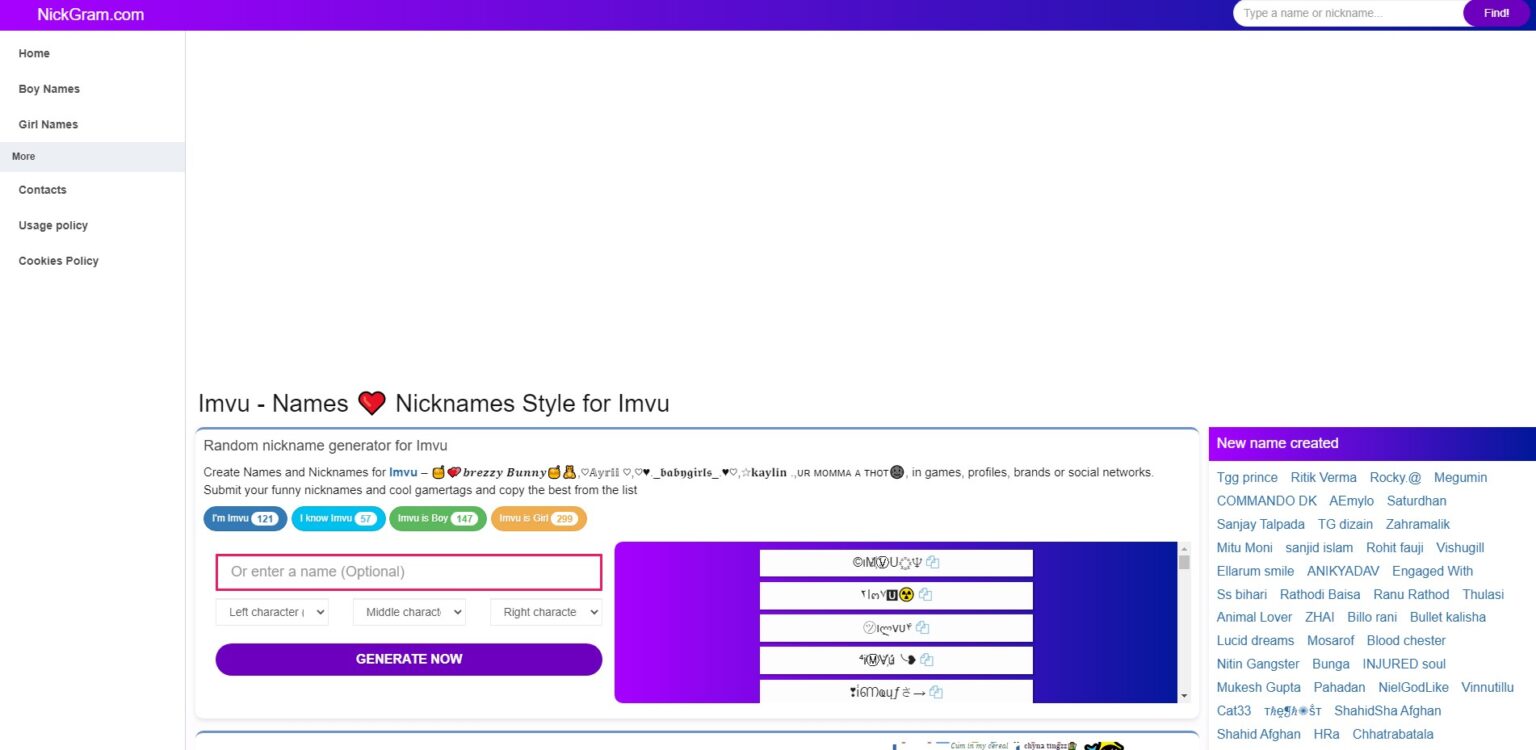This is an image capturing the homepage of the website nickgram.com. The top of the webpage features a header with a striking purple-to-blue ombre gradient, displaying the website’s name "nickgram.com" in bold white letters. Centered within this header is a search bar prompting users to "type a name or nickname," accompanied by a "Find" button.

The main body of the screen has a clean white background. On the left side of the screen, there's a vertical menu. The menu options include: Home, Boys Names, Girls Names, and More. The "More" option is selected, indicated by its slightly greyed-out appearance. Under the "More" category, there are subcategories listed: Contacts, Usage Policy, and Cookies Policy.

Beneath the header, the upper half of the white space is left blank. The lower half of the screen contains text related to IMVU. It mentions "IMVU Names" with a heart emoji, followed by "Nickname style for IMVU." Below this, there's a mention of a "Random Nickname Generator for IMVU," encouraging users to create names and nicknames for IMVU with example names like Breezy Bunny, Babgirls, Kaylin, Your Mama, and Thought in games, profiles, brands, or social networks. Instructions to submit funny nicknames and copy the best from the list are given. Additional options for submission are labeled "I’m Emu, I know Emu, Emu is boy, Emu is girl." There is also a prompt to enter a name and generate it.

Adjacent to this section, on the right-hand side of the screen, is a display filled with various characters and emojis, set against a blue-to-purple ombre background. At the far right, there is a section labeled "New Name Created," where a variety of newly generated names are presented.